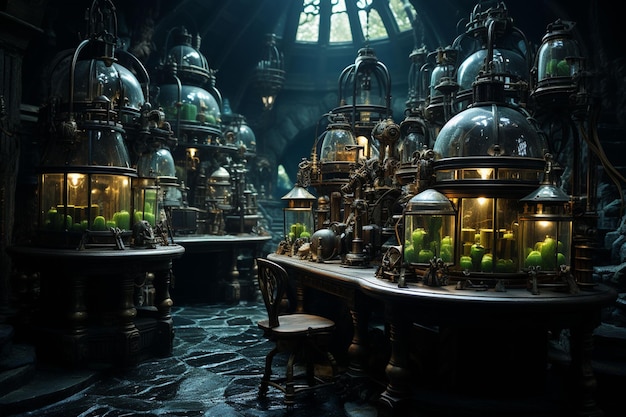The scene appears to be a computer-generated rendering set in a dimly lit, highly-stylized laboratory with a dark and mysterious ambiance. The room features a dark color palette dominated by dark mahogany tones and a black stone floor, possibly marble. The sparse lighting comes from a skylight above, resembling church-like windows, and a few hanging lanterns whose globes emit a subtle, possibly electric light. In the center of the room is a wooden chair facing a large table, surrounded by several other tables scattered throughout the space. These tables are adorned with numerous glass containers that have metal trims, resembling round terrariums or aquariums. Inside these containers are green, enigmatic objects that emit a soft glow, reminiscent of Granny Smith apples or candles. Additional small instruments and tools clutter the tables, contributing to the room's eclectic, almost steampunk atmosphere. This laboratory evokes an apothecary or wizard’s space, filled with arcane gadgets and mysterious green light.